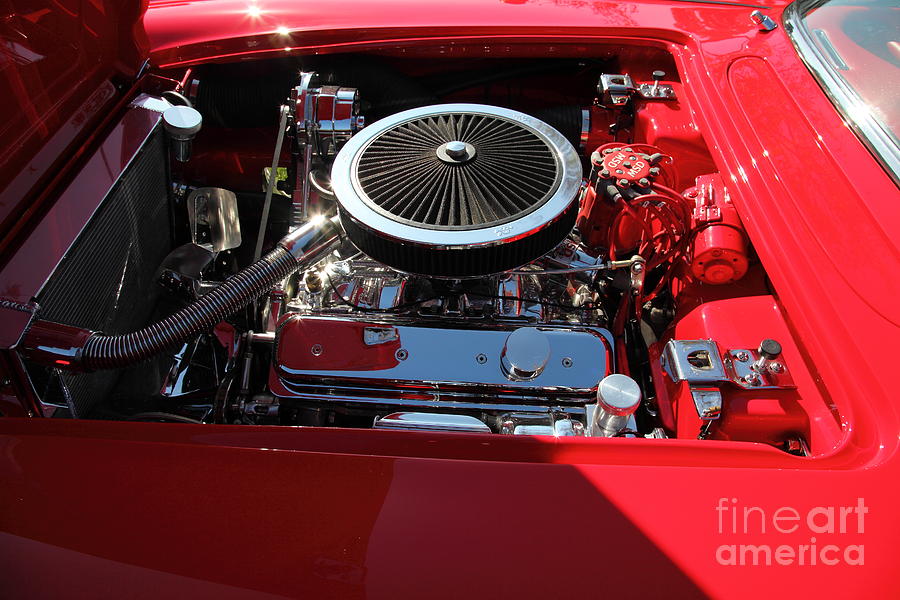This stunning image captures an impeccably restored antique car, resplendent in a vivid candy caramel red hue. Every detail of this classic automobile has been meticulously refurbished, from the gleaming metal finish to the pristine engine components. The viewer's focus is drawn to the car's engine bay, spotlighting a polished radiator and an eye-catching round silver element capped with a sleek black cover. Each piece of machinery shines with a freshly minted luster, indicating a thorough and loving restoration. The lower right-hand corner is subtly marked with "Fine Art America" signifying the image as a piece of art. This antique vehicle, while maintaining its timeless elegance, boasts a brand new interior and meticulously detailed undercarriage, epitomizing a perfect blend of vintage charm and contemporary perfection.